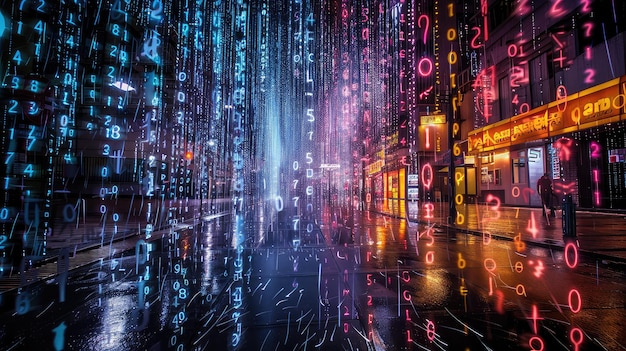In this detailed nighttime photograph, a futuristic cyberpunk city street is illuminated by a mesmerizing array of bright neon colors—cyans, pinks, purples, and reds. The scene, digitally rendered with a stylish touch, features numbers and letters streaming vertically from top to bottom, reminiscent of the iconic Matrix code. These symbols are predominantly blue on the left side and pink on the right, intermixed with the occasional letter, creating a holographic effect. The street itself is wet, glistening with puddles that reflect the vibrant lights from various businesses, whose illuminated signs suggest their varied statuses. On the right side of the image, a building adorned with bright yellow lettering catches the eye, though its purpose remains indistinguishable. The left side of the street is darker, highlighted by a lone fluorescent light. The street is mostly empty, save for a solitary figure walking with their head down by the neon-lit businesses. The overall atmosphere is one of eerie beauty, combining technological motifs with a noir aesthetic.